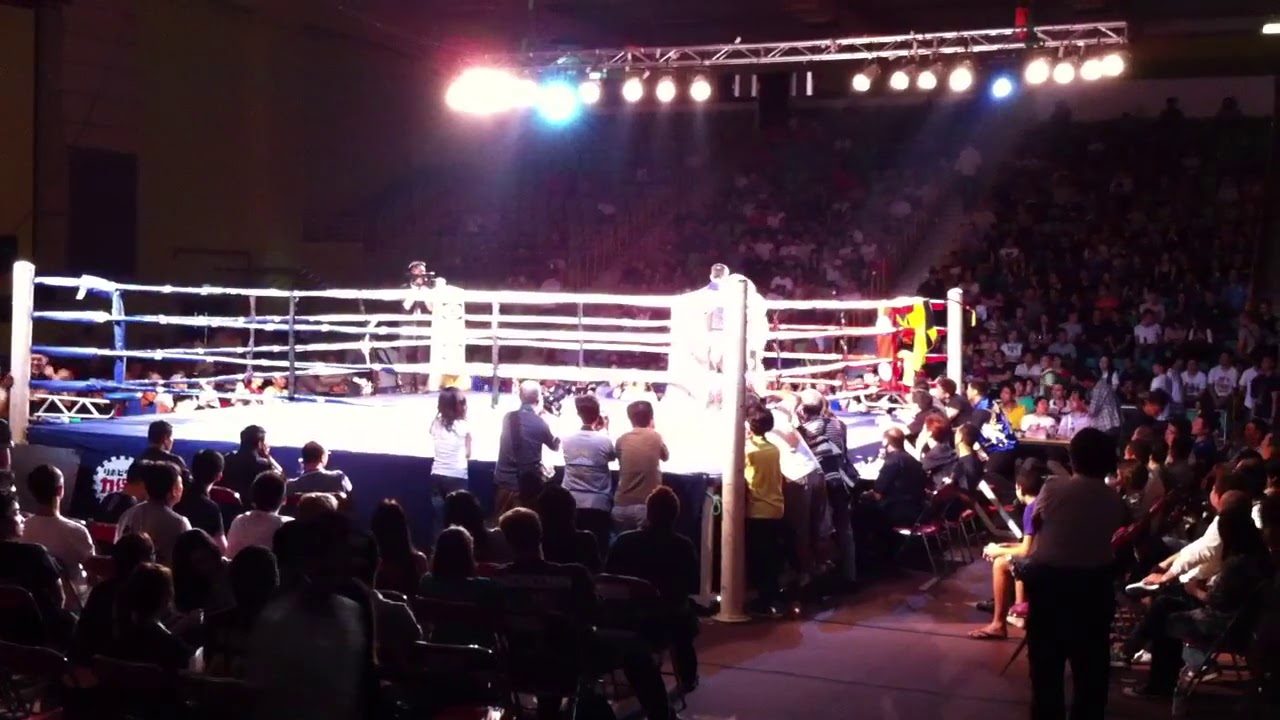The image captures an indoor wrestling ring, prominently featuring blue and white ropes and corner poles, illuminated by bright lights from a metal grid above. The ring sits at the center of a packed auditorium, with spectators filling tiered seating extending into the distance. Many attendees are seated in red chairs around the ring, some seated close by while others stand near the edges, observing intently. An announcer is present in the ring, wearing a robe, adding to the scene's lively atmosphere of a wrestling match. Bright lights reflect off the ring, highlighting the intense, competitive energy. The dark surroundings of the auditorium contrast with the well-lit ring, drawing focused attention to the action happening within.